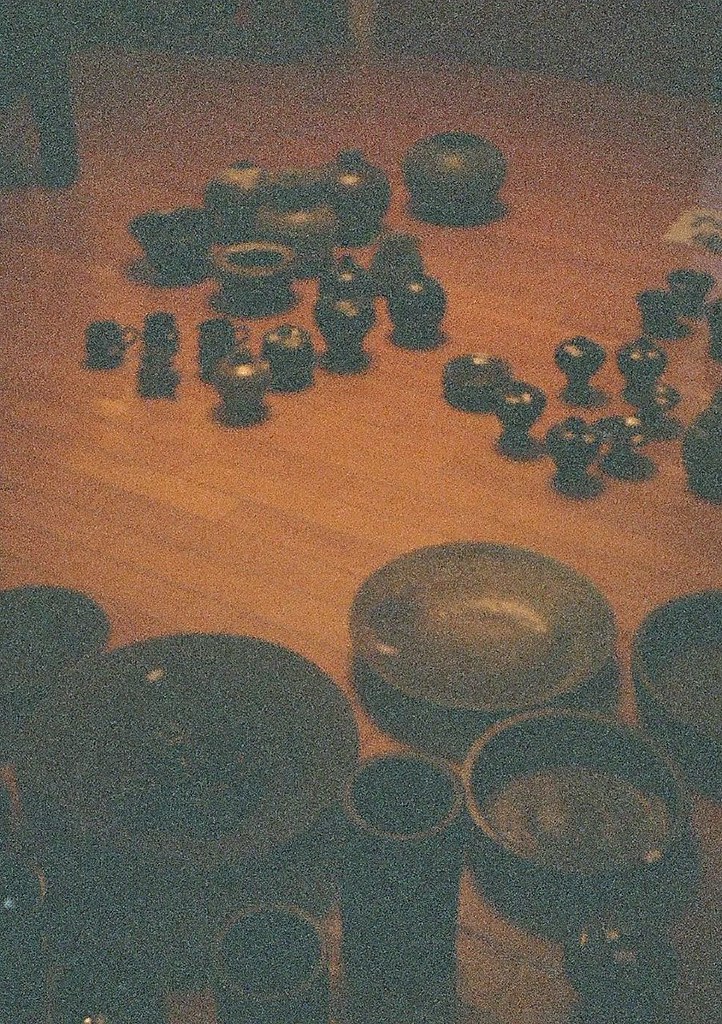The image is a grainy, somewhat dimly lit photograph depicting a collection of dishware arranged on a medium brown wooden floor, whose boards run diagonally from approximately 10 o'clock to 4 o'clock. In the bottom 40% of the photo, there's a grouping of dark-colored plates, bowls, and cups—ranging from black to possibly dark blue, green, and even some brown hues—arranged in a roughly three-to-four across by two-to-three high pattern. In the middle section, there’s a bare stretch of floor, providing a clear separation between the foreground objects and the items in the background. The upper section of the image features smaller objects, including tiny teacups, cup-like shapes with tiny lids, and bulbous vases with skinny necks and flared bases, which may be used for holding incense or sauces. Towards the top right corner, the leg of a chair is barely visible, partially obscured by the shadows.